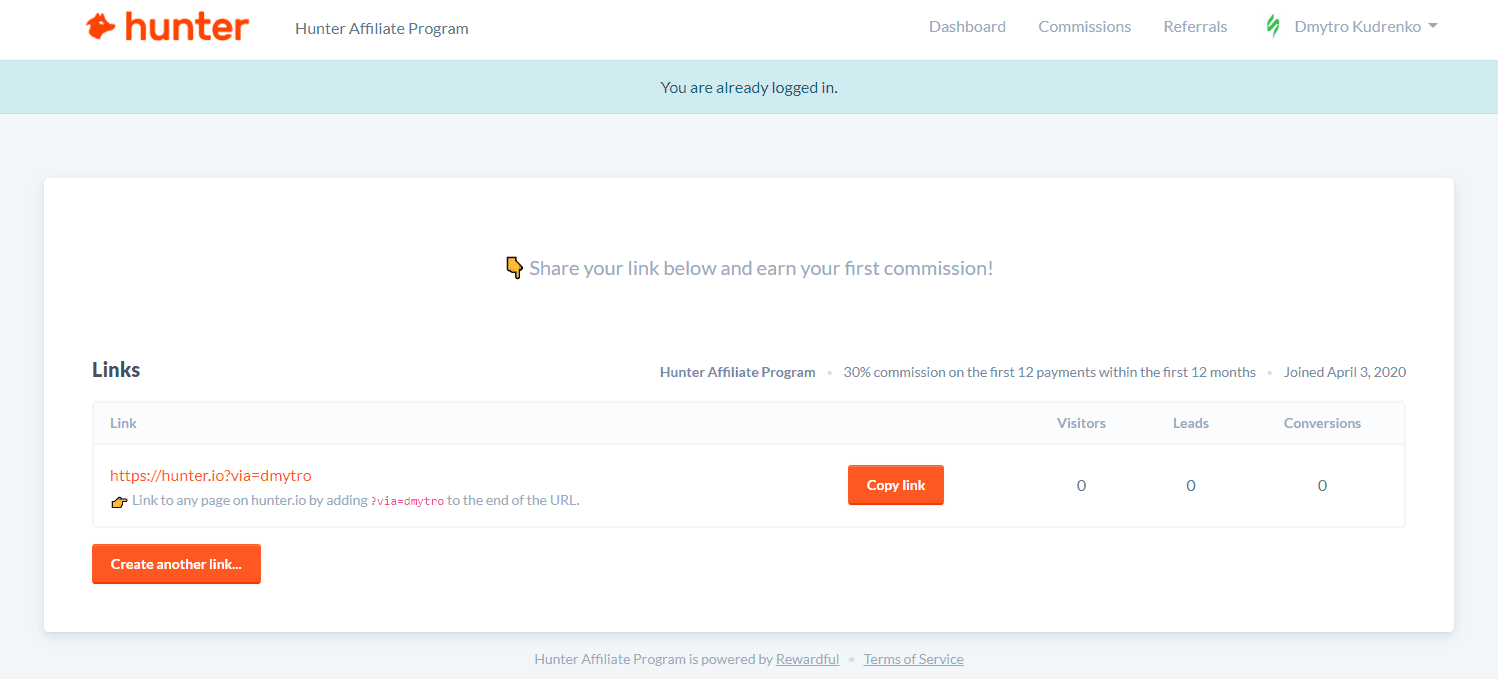The image showcases a webpage titled 'Hunter,' featuring a sleek design with a fox icon in red on the left-hand side, symbolizing the Hunter brand. The header of the page reads 'Hunter Affiliate Program' with navigation options listed to the right, including 'Dashboard,' 'Commissions,' and 'Referrals.' Also displayed is the user's name, Dimitri Kudrenko, marked by a small green icon beside it.

At the very top of the page, a prominent blue banner announces, "You are already logged in." Below this, the main content urges users to "Share your link below and earn your first commission," accompanied by a small illustration of a hand pointing downward. On the left side, there's a section labeled 'Links,' providing details about the Hunter Affiliate Program, which promises a 30% commission on the first 12 payments within the first 12 months. Additional information includes the user's join date, April 3, 2020.

Following this, there are columns for 'Visitors,' 'Leads,' and 'Conversions.' A specific, user-generated URL is highlighted in orange, along with an instruction to link to any page on hunter.io by adding a specific part of the website to the end of the URL. An orange 'Copy Link' box is prominently featured for easy copying.